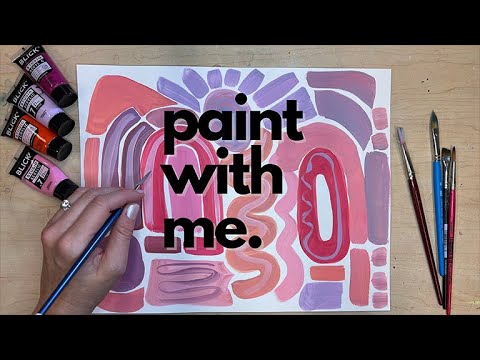The image appears to be a promotional screenshot from a potential online or YouTube painting class. It features a light wooden desk with a white sheet of paper in the center. A left hand, adorned with a ring and white pearl fingernail polish, holds a blue pencil over the paper. The paper is decorated with various colorful patterns, including squiggly lines, O's, half suns, slanted circles, zigzags, and spots, painted in shades of purple, orange, red, pink, and brown. To the left of the hand are four paint tubes in dark purple, light purple, red, and pink. On the right side, there are four paintbrushes and an additional pencil. The entire scene is framed by black borders at the top and bottom of the image, and prominently displays the text "paint with me." in large black lowercase letters.